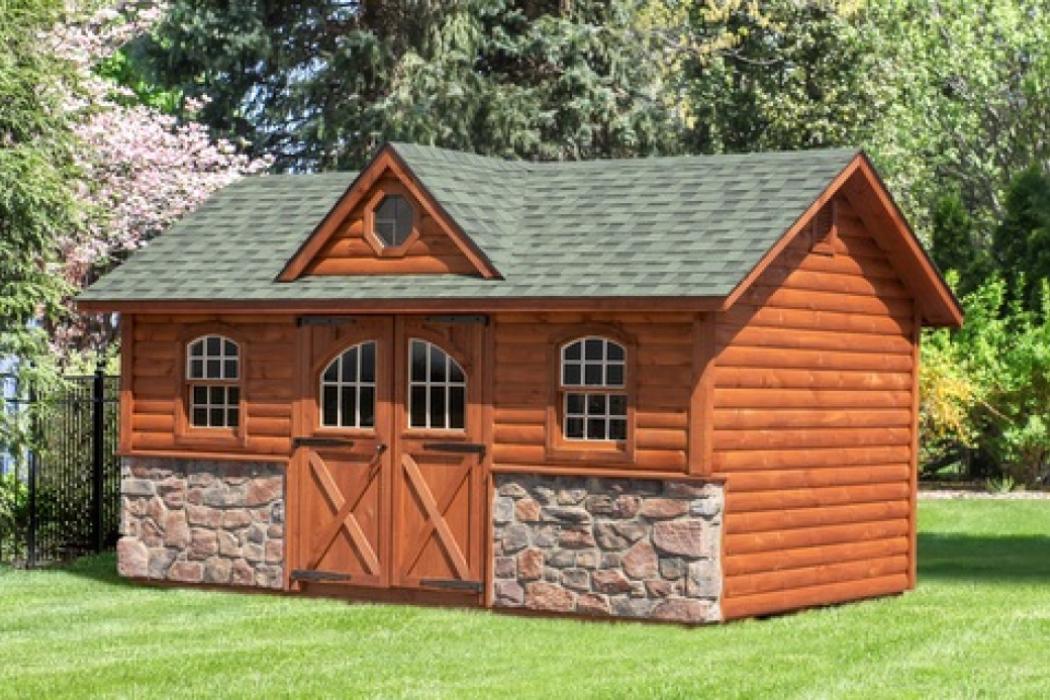The image depicts a rustic, small log cabin or shed set in a lush green garden space, surrounded by towering trees and bathed in daylight. The structure features a distinctive double door styled like barn doors, with windows embedded in them, and is crafted from light brown logs, though some describe it as having a red-stained appearance. A stone or brick facade accents the lower half of the cabin, adding a sturdy, charming element to its appearance. A window is positioned above the doors, suggesting a small attic area, and additional windows flank the main entryway. The cabin is topped with a v-shaped shingled roof, completing its quaint yet robust design. In the background, the tall trees include a mix of pine and leafy varieties, further enhancing the picturesque setting of this peaceful outdoor scene.